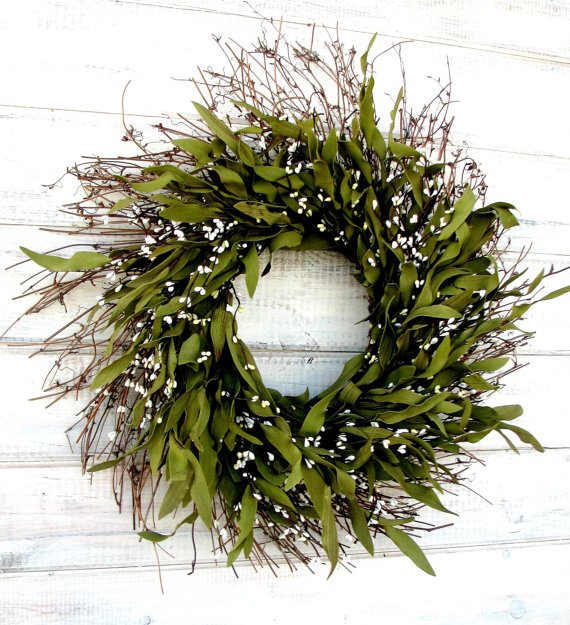This photograph showcases a detailed close-up of a green Christmas wreath against a backdrop of rough, aged white wooden slats. The wreath is composed of green leaves, brown twigs, and very tiny white flowers or bulbs scattered throughout. The leaves appear to be arranged in a counterclockwise pattern, giving the foliage a swooshing, dynamic feel. The wreath itself is rather unruly, with branches sticking out haphazardly, particularly at the top. The wreath takes up most of the image, and through its center, the white wooden slats are visible, some showing patches of blue and light brown, adding to the rustic charm of the scene. The weathered texture of the wooden slats and the glare on the right side of the wreath contribute to the overall aged and homey ambiance.